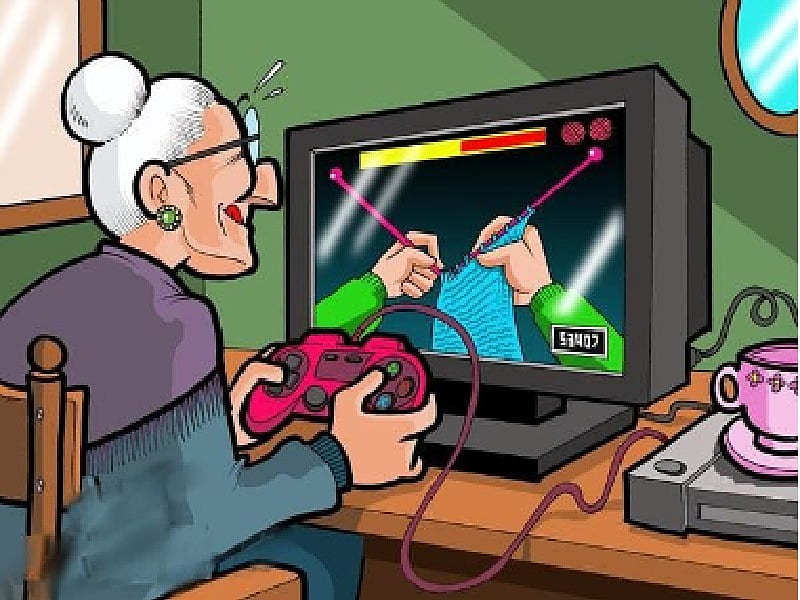The image is a highly pixelated, cartoon-like digital artwork reminiscent of a video game. It depicts an older woman, resembling a typical granny, with white or gray hair pulled into a tight bun. She is adorned with green earrings and a purple and blue shawl. She is holding a pink PlayStation-style controller that connects to a console on her right. The console, which resembles a PlayStation, has a pink teacup resting on top of it. 

The granny is seated in front of a TV screen that displays a video game, but instead of typical gameplay, the screen shows two hands engaged in knitting with large knitting needles. The room she is in has green walls adorned with nondescript photo frames. Her concentration is palpable, with her tongue sticking out to the right and a couple of cartoon sweat beads drawn on her forehead, highlighting her intense focus as she plays the knitting game.